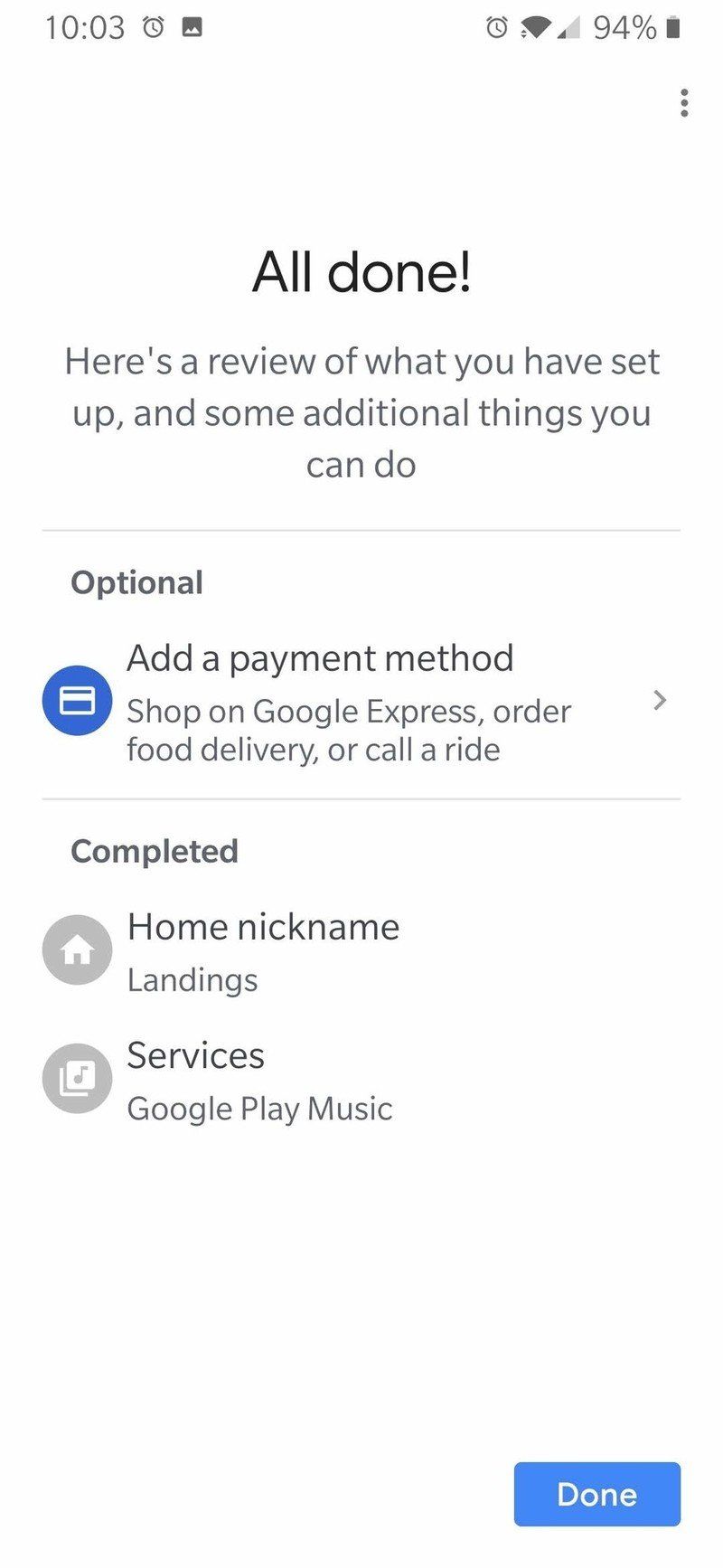The upper left corner of the screen is white, transitioning to gray. The time displayed is 10:03. Additionally, there is a long clock icon and a gray box featuring a zigzag white line. Another long clock icon is visible in the same gray hue. The Wi-Fi signal is shown as full, but the phone reception is low, also gray. The battery is charged at 94%.

Below this, there are three vertically aligned gray circles. The text "All done!" is prominently displayed in bold black lettering. Beneath this, in standard black font, reads, "Here's a review of what you have set up, and some additional things you can do." A thin gray line spans the width of the screen.

The word "Optional" appears in gray text. Adjacent to it is a blue circle containing a white card icon, accompanied by the text "Payment method." Further instructions suggest to "Shop on Google Express or order food delivery or call a ride." A gray arrow points to the right from here.

Another thin gray line separates this section from the next. The word "Completed" appears, followed by a gray circle with a white house icon, labeled "Home nicknames" in black text. "Landon's" is listed underneath.

Next, there is another gray circle with a white square and a gray music note inside it, labeled "Services" beside it. "Google Play Music" is written underneath.

At the bottom, a blue rectangle with white font states "Done" with a capital 'D'.